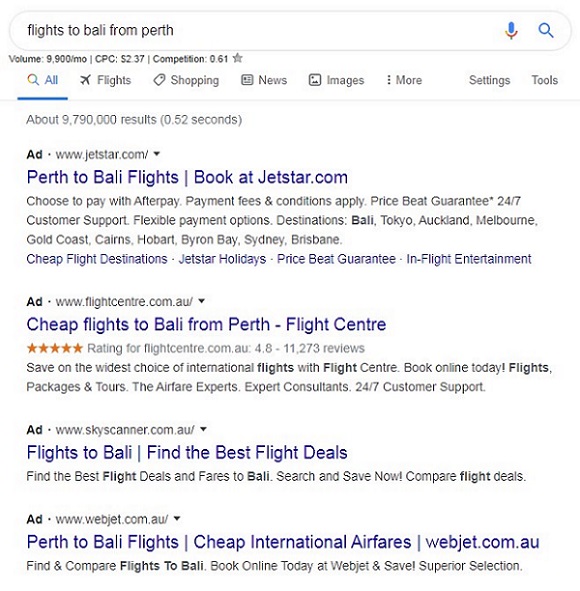In this image, a Google search bar displays a query for "flights to Bali from Perth." Below the search bar, there are four sponsored URLs, highlighted as advertisements.

1. **Jetstar.com:**
   - **URL Description:** "Perth to Bali flight - Book at Jetstar.com" (displayed in blue text)
   - **Detailed Description:** "Choose to pay with Afterpay. Payment fees and conditions apply. Price Beat Guarantee, 24/7 customer support, and flexible payment options available. Destinations include Bali, Tokyo, Auckland, Melbourne, Gold Coast, Cairns, Hobart, Byron Bay, Sydney, and Brisbane."
   - **Additional Links:** "Cheap Flight Destination," "Jetstar Holidays," "Price Beat Guarantee," and "Inflight Entertainment" (all links in blue).

2. **FlightCenter.com:**
   - **URL Description:** "Cheap Flights to Bali from Perth - Flight Center"
   - **Detailed Description:** "Save with the widest choice of international flights. Book online today. Offering flights, packages, and tours. Consult with airfare experts. 24/7 customer support. This website is rated 4.8 stars by 11,273 reviews."

3. **Skyscanner.com.au:**
   - **URL Description:** "Flights to Bali - Find the Best Flight Deal"
   - **Detailed Description:** "Find the best flight deals and fares to Bali. Search and save now. Compare flight deals."

4. **Webjet.com.au:**
   - **URL Description:** "Perth to Bali Flight - Cheap International Airfares - Webjet.com.au"
   - **Detailed Description:** "Find and compare flights to Bali. Book online today at Webjet.com.au and save. Superior selection of flights."

Each option offers unique selling points and various features to help travelers find and book their flights conveniently.